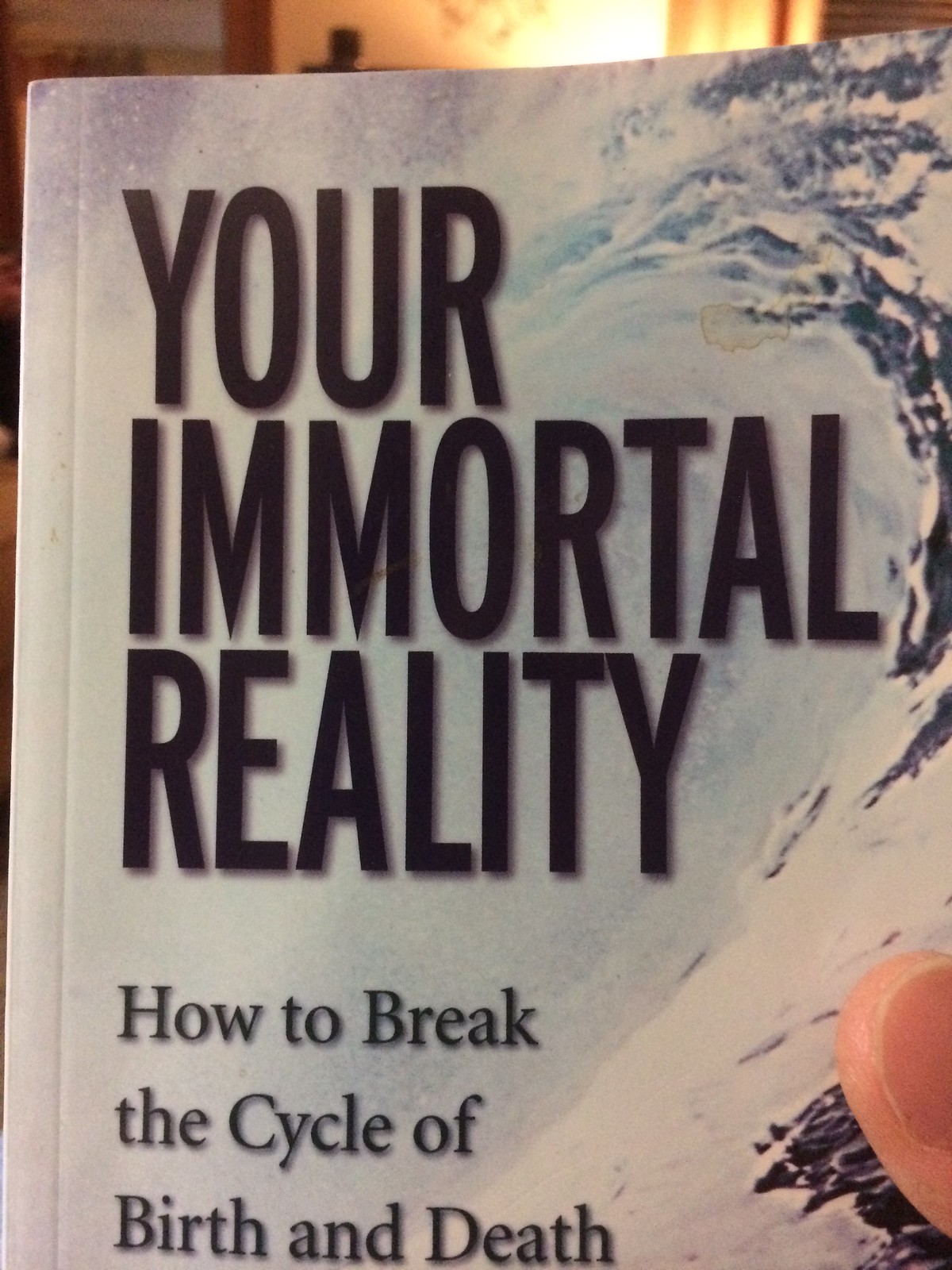This image depicts a close-up of the front cover of a book titled "Your Immortal Reality: How to Break the Cycle of Birth and Death." The book features a dynamic design with an ocean wave as the primary background, exhibiting hues of light blue with white accents, giving it a swirling, powerful appearance. A person's thumb and fingernail are visible, holding the book on the right-hand side. There's a narrow strip around the top and side, suggestive of the book being within an indoor setting, possibly near a window with sunlight streaming through. An additional detail includes a small coffee stain in the upper right corner of the cover, adding to the realism of the scene. The left side of the book shows a visible crease where it would open, hinting at the start of the pages inside. The background is mostly focused on the book itself, with the light from outside providing subtle illumination.